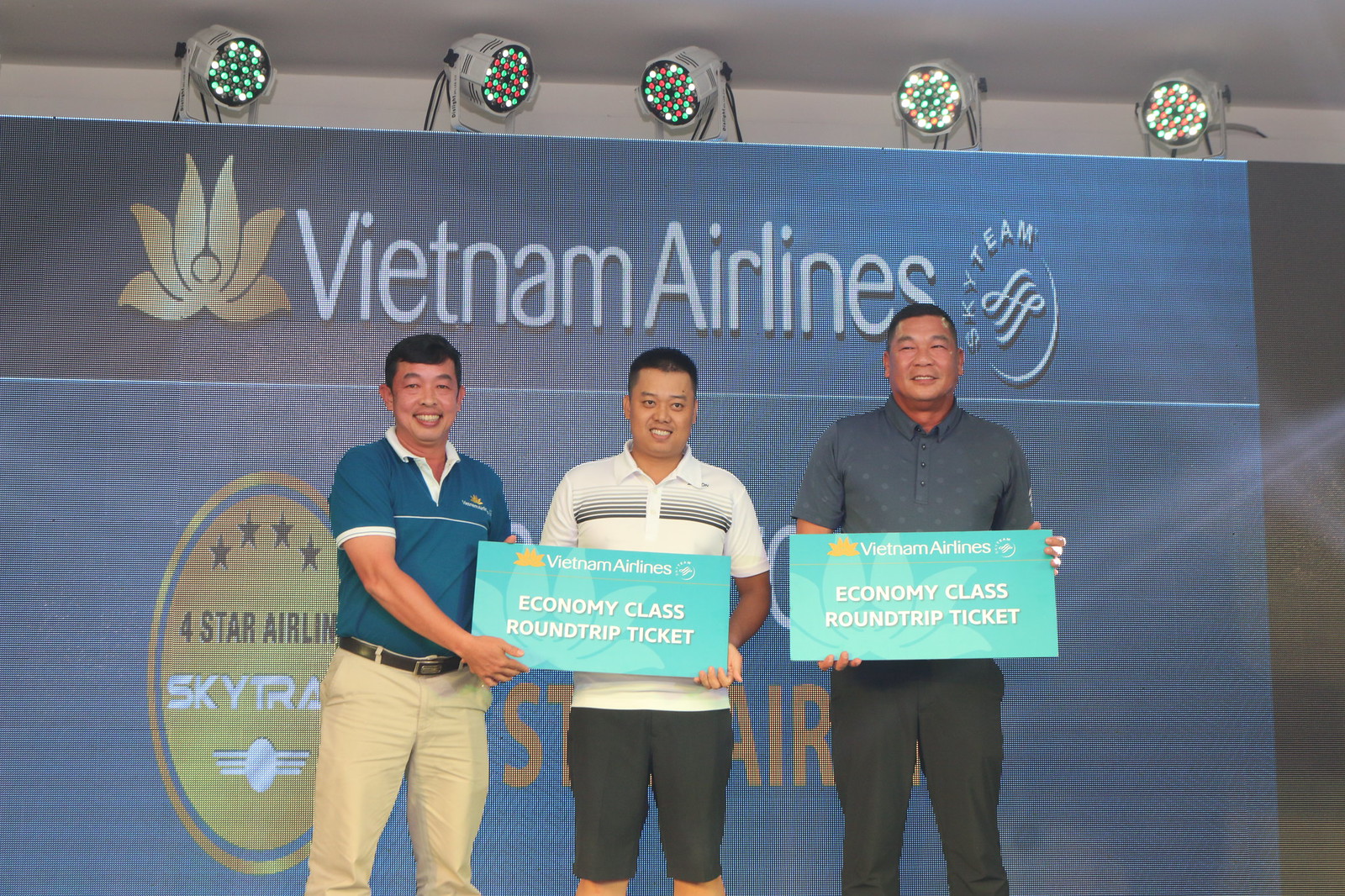In an indoor setting, this photograph captures three men standing and smiling in front of a large blue banner adorned with the white text "Vietnam Airlines" and a gold lotus flower logo to the left, indicating a Four Star Airline rating. The banner is further embellished with multi-colored spotlights from a white ceiling. Each man holds a rectangular green board that reads "Vietnam Airlines Economy Class Round Trip Ticket." On the left, a man with short black hair, wearing a teal shirt and khaki pants, shares the board with the middle man, who has short black hair and is dressed in a white polo shirt featuring black stripes and black knee-length pants. The man on the right, in a gray shirt and gray pants, holds his own matching ticket. The vibrant backdrop and their unified poses suggest a celebratory or promotional event.